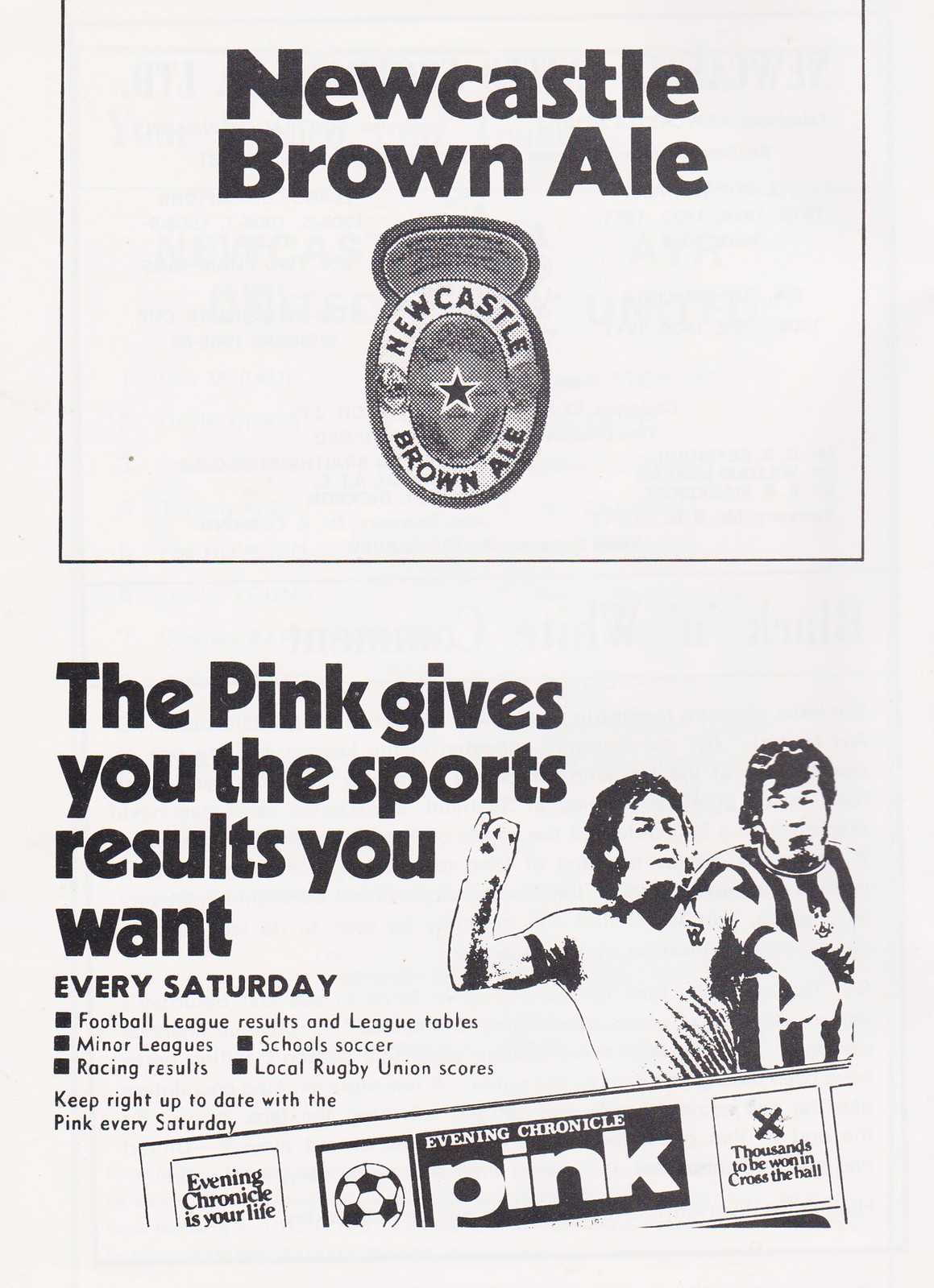This is a vintage advertisement flyer promoting Newcastle Brown Ale, prominently featuring the bold and dark font of the brand's name alongside its iconic logo with a star in the center. Below the Newcastle Brown Ale branding, the flyer transitions into an advertisement for the Evening Chronicle’s special Saturday edition, referred to as the "Evening Chronicle Pink." This section, outlined by a black border, emphasizes in bold black text that "The Pink gives you the sports results you want every Saturday," and details the variety of updates offered, such as football league results, minor leagues, racing results, school soccer, and local rugby union scores. The flyer encourages readers to "keep right up to date with the Pink every Saturday," and asserts that "Evening Chronicle is your life." Enhancing the sporty theme, there is a picture of two men, appearing to be a referee and a player, as well as an image of a soccer ball. Additionally, the flyer mentions, "thousands to be won in cross the hall," further enticing readers.